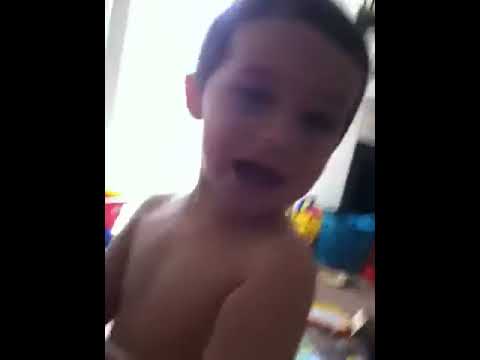In this photo, we see a young boy, around two to three years old, with brown hair. He appears to be in motion and looking directly at the camera, his mouth open as if caught mid-laugh. The boy is bare-chested, possibly just out of the bath, with a towel draped across one of his shoulders. He stands in the center of a room, likely a playroom, with various objects and toys scattered around him. To his left is a toy pushing cart, while to his right are blue storage baskets for the toys, positioned near the opening of what looks like a fireplace. The setting is indoors during the day, with light streaming through a window behind him, enhancing the warm, playful atmosphere of the scene. The colors in the image include off-white, white, black, tan, yellow, red, blue, and brown.